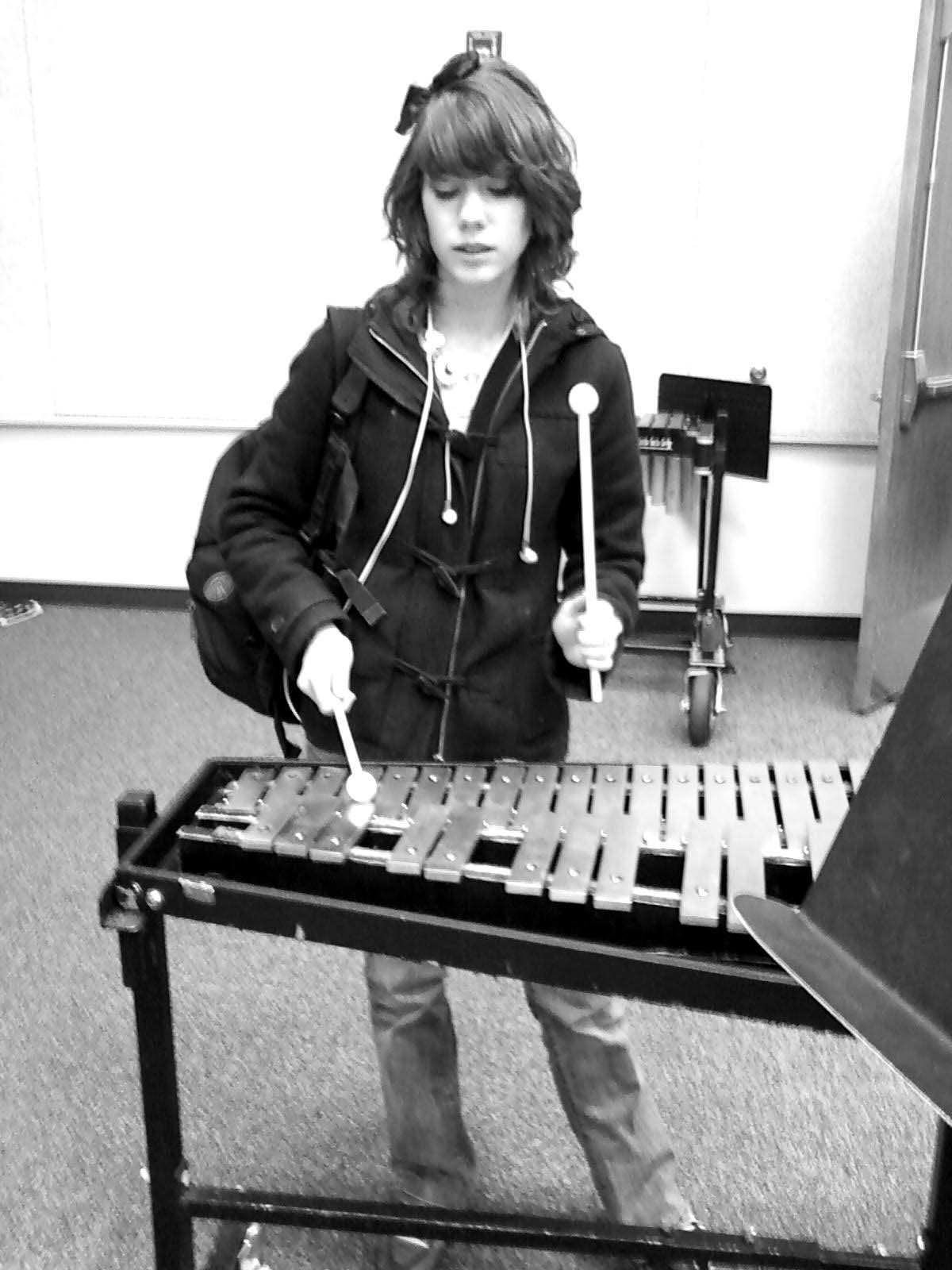This black and white photograph captures a young woman, possibly a student, deeply engrossed in playing a xylophone. She is wearing a black coat with a hood, though the hood is down. A backpack is slung over her right shoulder (our left) and she sports blue jeans. Her short, wavy, shoulder-length hair, styled in layers with bangs, features a bow adorning the right side of her head. With xylophone sticks in each hand, one stick is striking the instrument while the other is in mid-air. In the background, the setting seems to be a classroom, with another xylophone and a music stand visible. To the right, there's a glimpse of a wooden door slightly ajar and part of another music stand in the corner, all set against a carpeted floor. The sizeable xylophone takes center stage in the image, capturing the focus and dedication of the young musician.